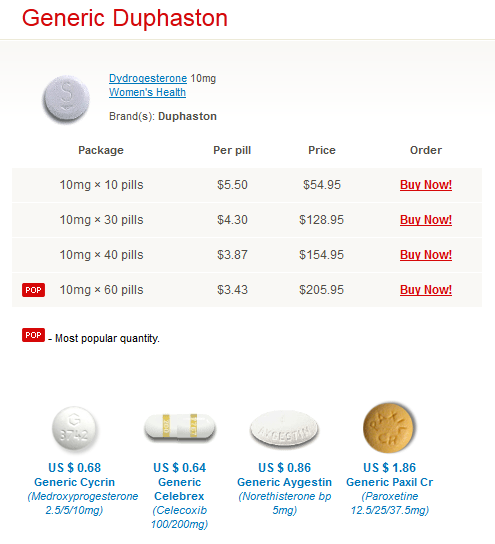The image depicts a detailed price chart for various generic medications. At the top is "Duphaston," a brand name for a synthetic hormone, indicated by the round pill shape. The chart lists the cost per milligram and is divided into columns detailing the price for different quantities—10, 30, 40, and 50 pills—including a "buy now" option.

Further down the image, there is a "most popular quantity" section, followed by images of different generic pills. One entry shows a pill costing $0.68 with the label "Generic Siren CYC" and a long chemical name indicating a type of progesterone. Another entry lists "Generic Celebrex," though the specific drug name is unclear. Other medications include "Generic Aigestin" and the more expensive "Generic Paxil CR," priced at $1.86. 

Overall, the image provides a comprehensive breakdown of pricing, quantities, and purchasing options for various generic medications, but does not elaborate on their specific uses or effects.